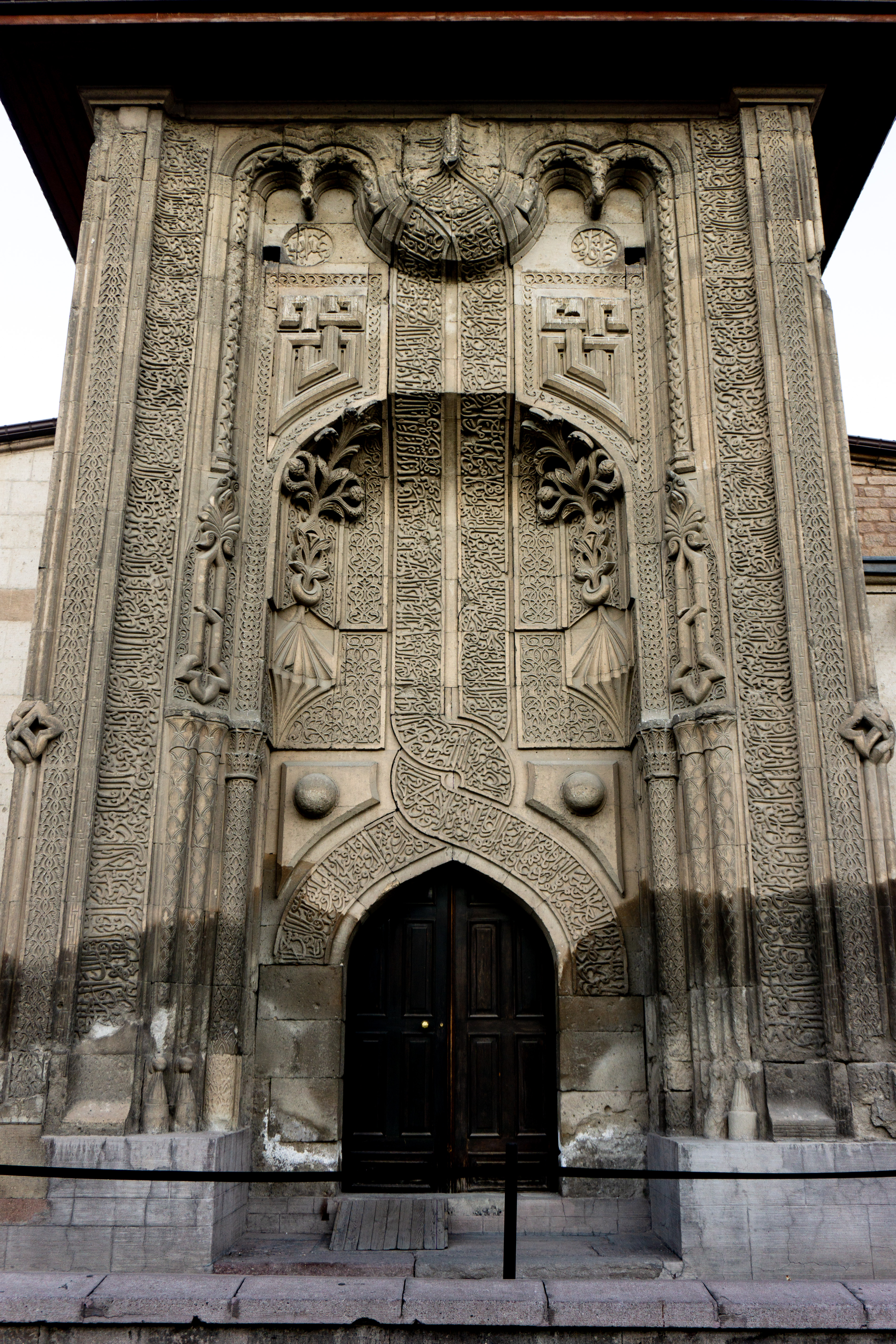This image features a historic, dark tan stone church or cathedral captured from across the street. Dominated by a tall, column-like entrance, the building exudes an old-world charm, reminiscent of European architecture. Intricate carvings embellish the façade, including vine patterns and fleur-de-lis at the top of the structure. The entrance boasts a pair of arched double doors, dark brown with golden doorknobs on the left side, framed by a dome-shaped overhang with a reddish hue. A gray concrete sidewalk leads up to a small set of steps and a gray wall flanking the entrance. Beneath the upper steps lies an old wooden pallet serving as a makeshift ramp. Encircling the entrance is a black security line, creating a subtle boundary between the sidewalk and the street. The background reveals a sky punctuated by clouds, adding to the timeless and serene aura of the building.